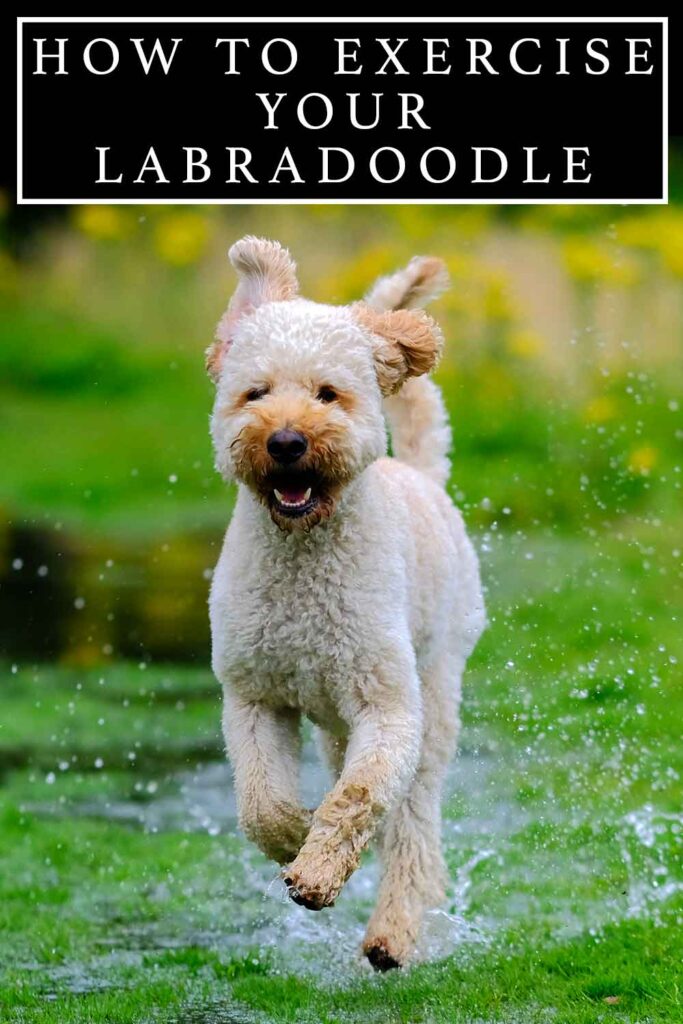The image features a lively young labradoodle with fluffy, cream-colored fur and distinctive tan markings around its nose, ears, and paws. The dog's black eyes and happy expression, with its mouth open and bottom teeth visible, convey its playful spirit as it runs joyfully through a large water puddle. Water droplets splash up around the dog, which stands on green grass, suggesting the puddle is part of a yard or common area. The dog's thick legs are in various positions, indicating motion, with its tail straight up in the air and ears flopping enthusiastically. Above the vibrant scene, the text "HOW TO EXERCISE YOUR LABRADOODLE" is prominently displayed in white capital letters on a black background, providing context for the energetic display. Bright yellow flowers are visible in the background, adding a touch of color to the natural setting.